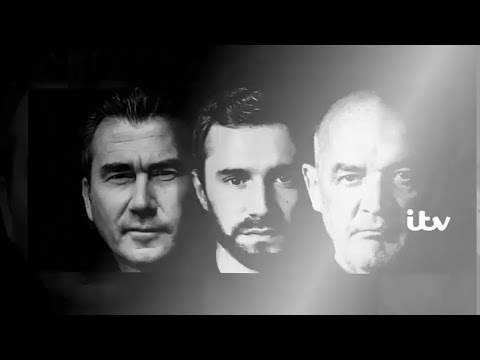In a dramatic black-and-white image, three light-skinned men are closely positioned next to each other, forming a trio against a highlighted background with sun rays emanating from the top right. The leftmost man appears to be an older gentleman in his late 30s, sporting short gelled-up brown hair, squinted eyes, and slightly swollen facial features. His face is partially shadowed compared to the others. The central figure is distinctly the youngest, likely in his early 20s, with dark, neatly styled hair swept from left to right and a short, well-groomed beard and mustache. His face is brightly illuminated. On the right stands an older man, comparable in age to the leftmost figure, with a bald head and messy, black eyebrows. His expression is set in a grimace, with one eye appearing slightly misaligned. His only facial hair is sparse stubble. Above and below their faces are black bars, and to the right of the rightmost man's cheek, the letters "ITV" are prominently displayed in white.